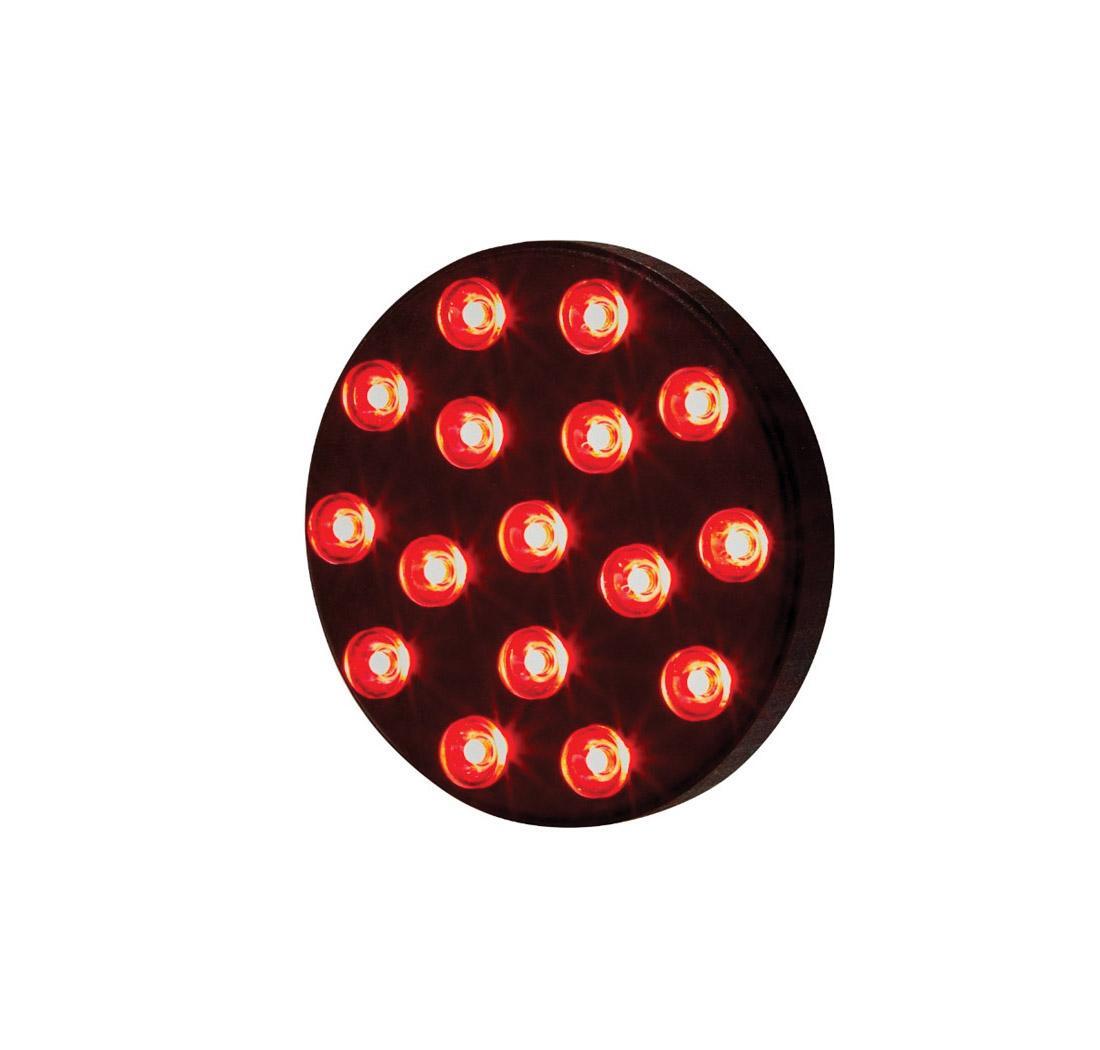The image features a flat, round black disc, possibly made of plastic, with no visible background, emphasizing the object itself. The disc, resembling some sort of utility or lighting device, is adorned with multiple red LED lights. These lights are arranged in a specific, almost circular pattern. The outermost ring comprises 16 red LED lights, while inner rings contain 10, and 5 lights respectively, with a single central LED light at the heart of the arrangement. The lights form various geometric patterns, including an impression of triangular groupings, and illuminate brighter at the center, fading slightly towards the edges. The detailed arrangement and illumination suggest this disc could be a specialized lighting fixture, possibly designed to be mounted on a ceiling or wall.